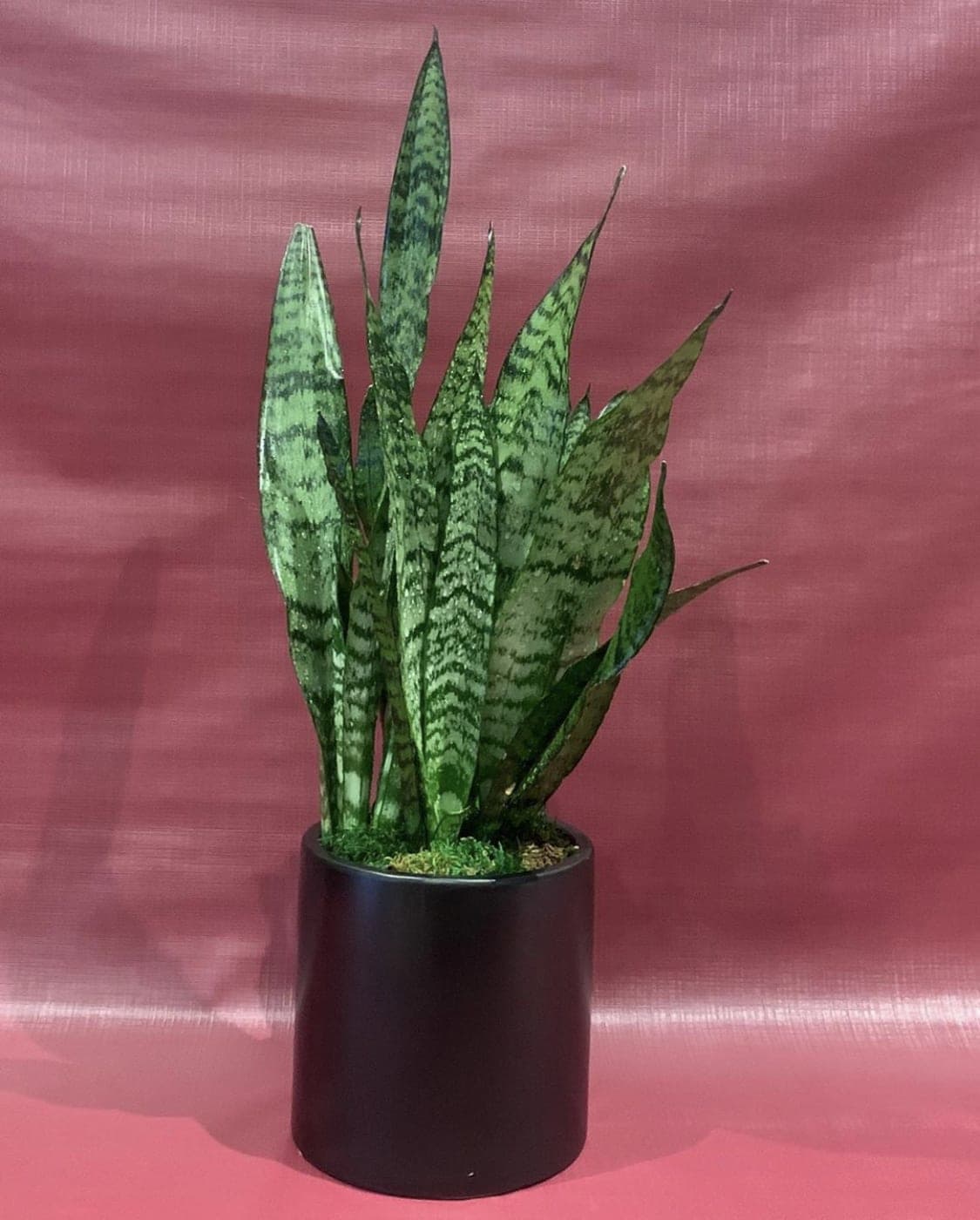This image showcases a house plant elegantly potted in a medium to large black cylindrical pot with a semi-shiny, satin-like finish. The top of the pot features a ground cover that is predominantly green with some yellow and darker hues, possibly shadows cast by the plant itself. The plant has tall, vertical leaves that emerge straight from the pot, displaying a mixture of dark and light green shades. There is a possibility that the plant is artificial, though it's indistinguishable from the image alone. The pot is placed on a burgundy-colored tarp that also wraps halfway up the wall behind it, providing a distinct backdrop that contrasts with the lush greenery of the plant.